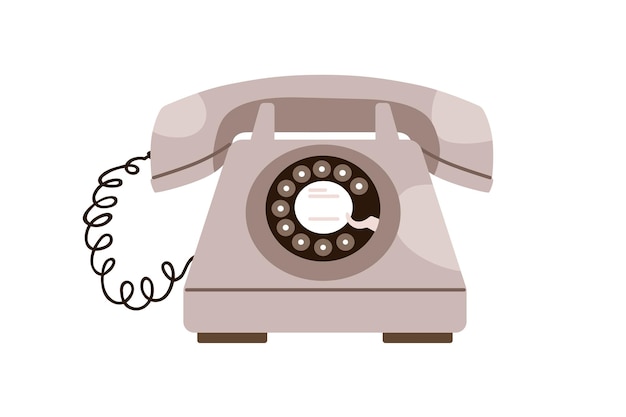This image depicts a minimalistic 2D graphic design of an old-timey rotary telephone set against a flat, plain white background. The telephone, centrally positioned in the illustration, showcases a light pinkish-brown hue with slight variations in tone to suggest texture. The base of the phone, shaped like a parallelogram, widens at the bottom and narrows towards the top, where two small protrusions act as supports for the handheld receiver. The phone's cord, depicted in a lighter gray shade, extends from the left side of the receiver to the base. Featuring a classic rotary dial, the front of the phone displays a white circle encompassed by a dark brown ring, containing smaller circles and a dialing hook for finger placement. Although there is some unreadable lettering within the central white circle, the overall design remains clean and simplistic, characterized by its flat appearance with no discernible shadows or dimensions. The illustration might resemble an icon, thumbnail, or emoji due to its stylized and minimalistic execution.